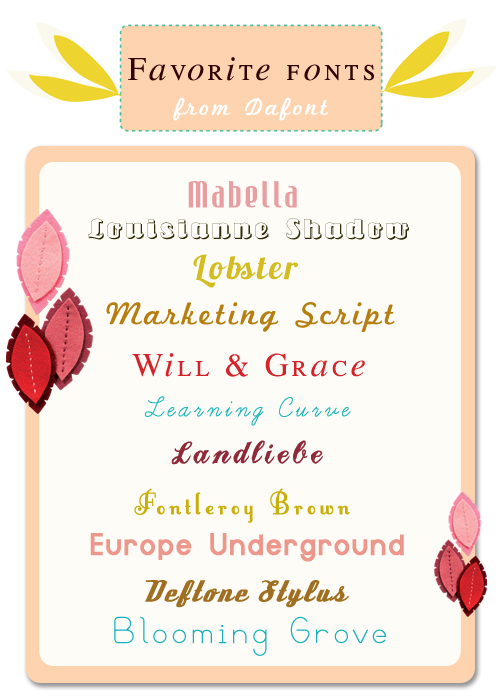The image is an advertisement showcasing a selection of favorite fonts available on DaFont. At the top center, within a peach-colored rectangle, the text "Favorite Fonts from DaFont" is displayed. The phrase "favorite fonts" is in a brown font, while "from DaFont" is in a white, cursive font. Flanking this central rectangle are two yellow leaves on either side. Below this, a larger rectangle bounded by a peach border encloses a white background displaying various font names in different colors and styles. These fonts include Mabella in pink, Louisiana in white with a black outline, Lobster in yellow, Marketing Script in brown, Will & Grace in pink, Learning Curve in sky blue, LandLieb in dark purple, Font Leroy Brown in dark yellow, Europe Underground in light pink, Deftone Styles in brown, and Blooming Grove in light blue. Adding to the visual appeal, the peach frame is adorned with clusters of three leaves in shades of pink, red, and crimson red at the top left and bottom right corners. The overall design combines these pastel and vibrant hues, creating an eye-catching and informative display against the white background.